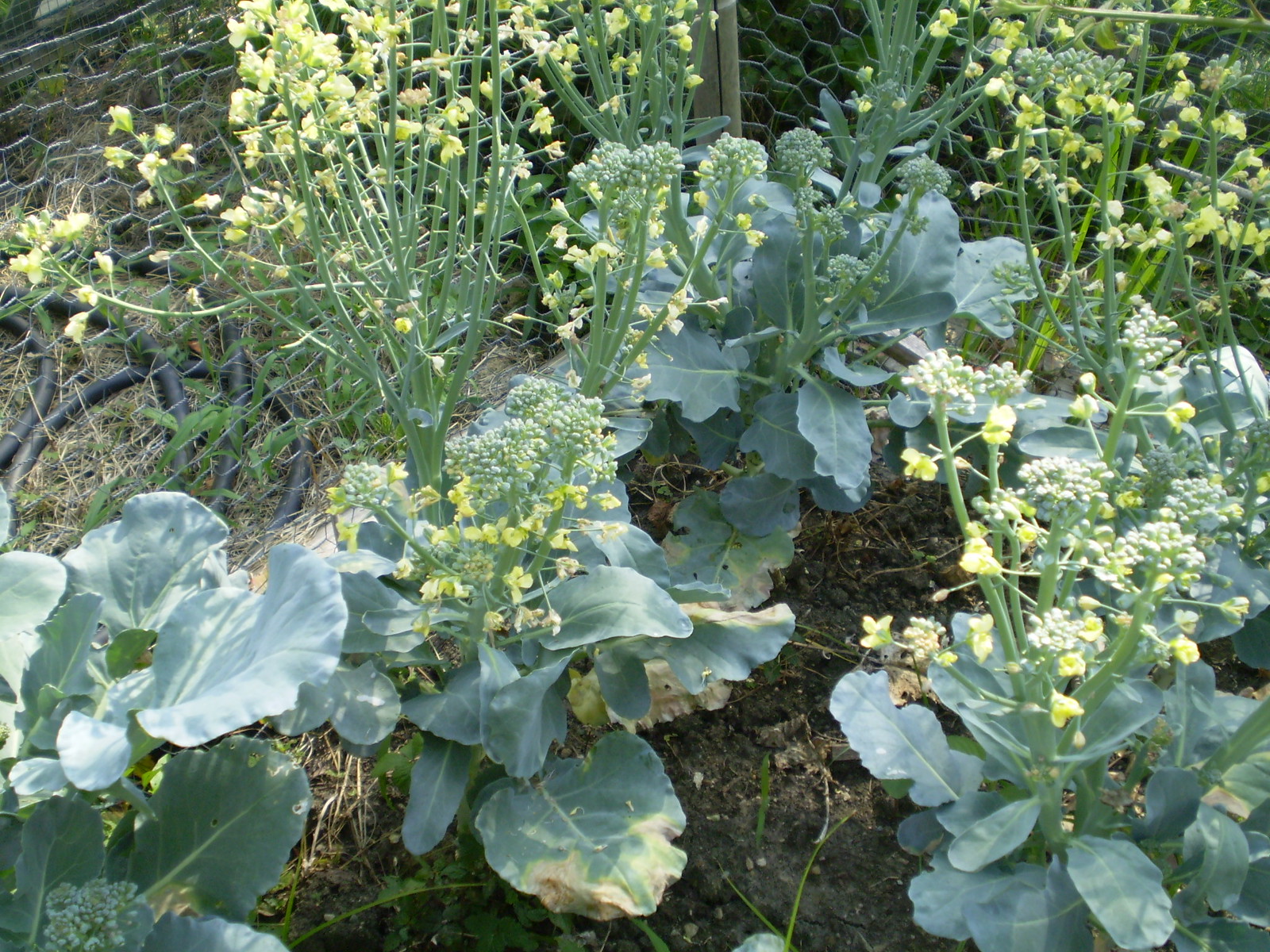This photograph captures a corner section of a simple garden with rich, dark brown soil. In the foreground, a cluster of wide, leafy green plants, potentially vegetables like collard greens or kale, are growing healthily despite their leaves appearing dusted with a powdered-like substance. Tall stems rise from these plants, crowned with small but detailed yellow flowers. The flowers are budding, with some blooms appearing greenish-yellow and others possibly white, indicating they may still be tight buds. Patchy grass is visible among the greenery. The background reveals a chicken wire fence angled at two sides, with a dark cable or hose running along the ground behind the mesh. This fence encloses the garden, hinting at its protective purpose for the vibrant plants within.